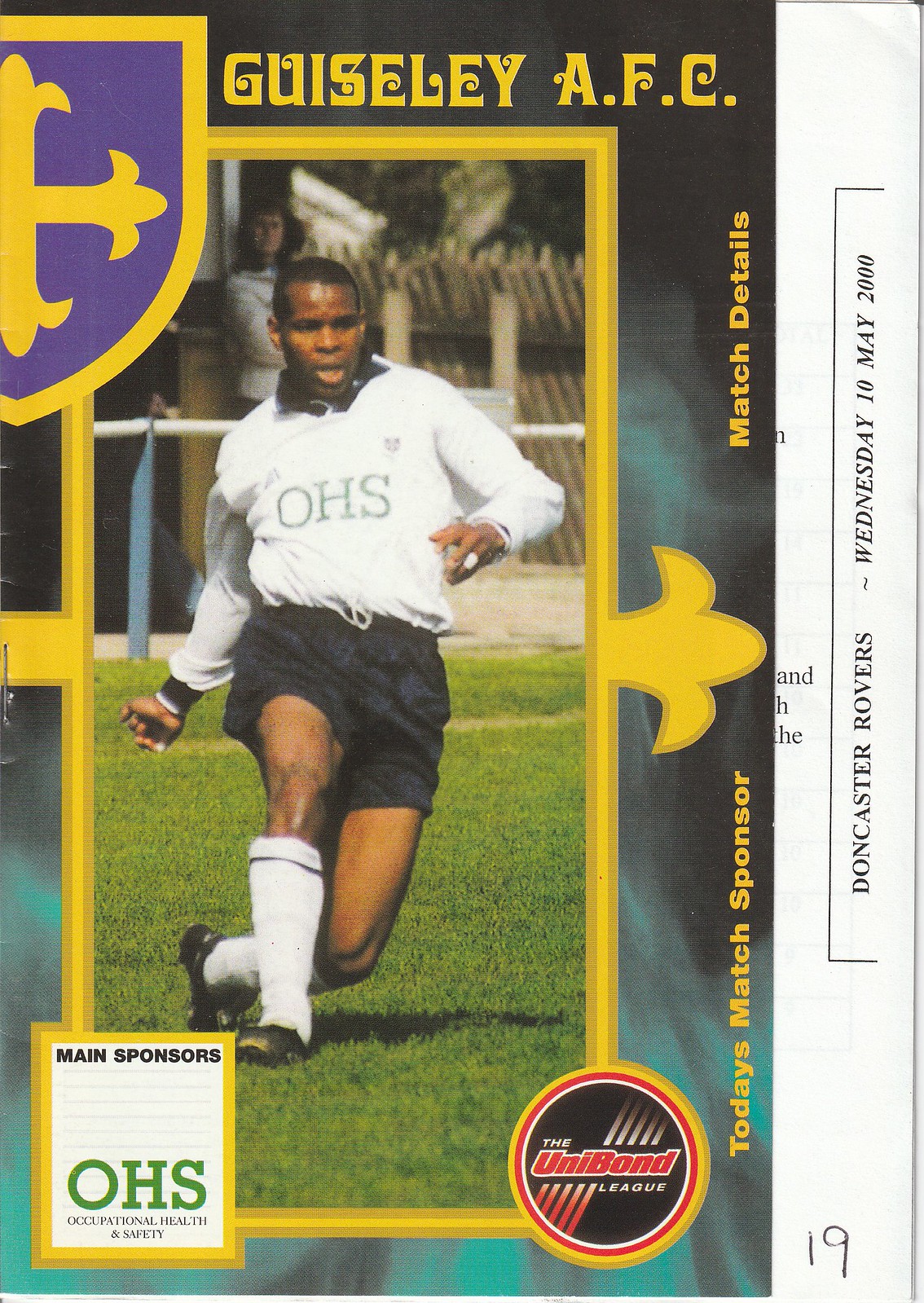The cover of this sports magazine or match program prominently features a dynamic photograph of an African-American soccer player. He is caught mid-stride with his left knee slightly bent, wearing black soccer cleats, tall white shin guards with a black stripe at the top, and short black silky shorts. His white long-sleeve jersey has black cuffs and a black collar, with "OHS" printed across the front, indicating his team’s sponsor is Occupational Health and Safety. He also has tape on some of his fingers. The left side of the image contains a column with black text reading "Doncaster Rovers, Wednesday, 10 May 2000," and a shield with a cross and floral designs, outlined in yellow. At the top, bold yellow text announces "Guiseley AFC." The right edge of the cover includes text stating "Today's Match Sponsor" and "Match Details," along with the Unibon League logo in a circle, and various other logos at the bottom.